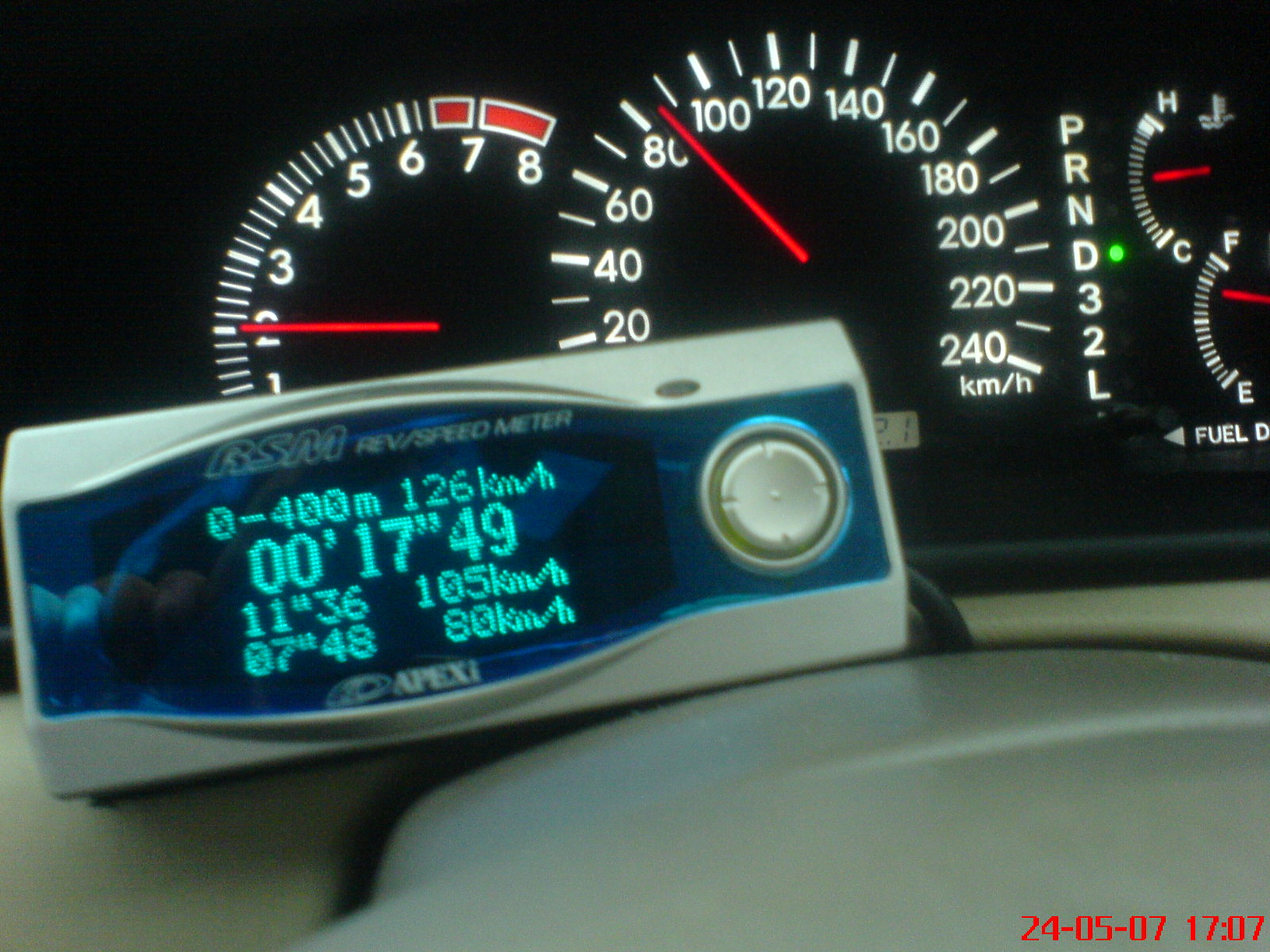A detailed close-up photograph of a car’s dashboard displays various gauges and indicators with precision. At the center, the speedometer prominently features a range from 20 km/h to 240 km/h, with a red needle currently pointing at 60 km/h. Adjacent to it, the RPM gauge spans from 1 to 8, with the red needle stationed at 2. In the lower right corner, red text indicates the date and time as "24 05 07" and "17:07."

A vertical indicator labeled "PRND 3 2 L" has a green light illuminating next to "D," signifying the car is in drive mode. The fuel gauge, marked from full to empty, shows approximately three-quarters full, while the coolant temperature gauge, ranging from H to C, is positioned at the midpoint.

Additionally, a white rectangular box with a blue interior provides detailed speed and distance data, displaying "RSM rev/speed meter 0 to 400 meters," "126 km/h," "1749," "1136," "105 km/h," and "748 80 km/h."